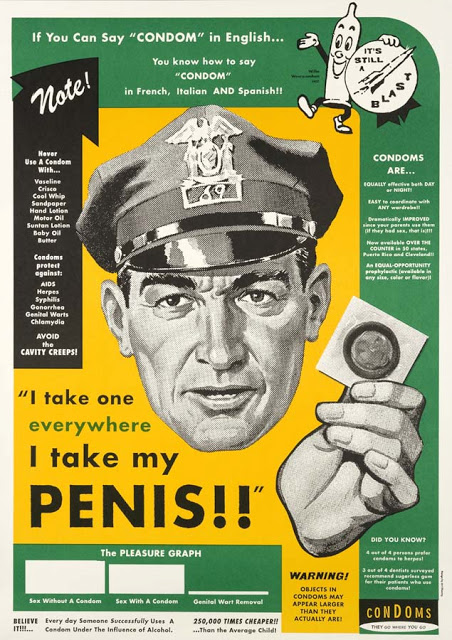This vintage-style advertisement poster, resembling a 1950s magazine illustration, humorously promotes condom use. Dominating the yellow-background frame is a detailed, black-and-white clip art of a retro-styled policeman, identifiable by his 50s-era uniform hat adorned with an eagle emblem and the number 69. The officer’s hand, shown in a detailed grip between thumb and forefinger, holds a packaged condom. Emphasizing the message below his stern visage in quotations is the cheeky slogan: "I take one everywhere I take my penis."

Detailed information borders the poster on three sides. At the top and along the green-edged right border, various condom-related facts are displayed in white font. A distinctive element in the upper right corner features a lively cartoon condom, its black arms and legs contrasted by white hands and feet, a broad smile on its face, and it holds a white circle with a ribbon, inscribed with "it's still a blast" alongside a rocket illustration.

On the left, bordered by a black vertical bar with an arrowhead top, detailed advice in white text warns against using condoms with substances like Vaseline, Crisco, and motor oil. It emphasizes condoms' protective benefits against sexually transmitted infections, listing AIDS, herpes, syphilis, and more.

Below the policeman’s headshot and slogan, a playful green bar graph labeled "the pleasure graph" dramatically illustrates the comparative enjoyment of sex with and without condoms, humorously ranking "genital wart removal" the lowest. At the bottom, additional comedic insights like "250,000 times cheaper than the average child" and "Warning: objects and condoms may appear larger than they actually are," amplify the poster’s humor and educational aim. The multifaceted, colorful design blends a nostalgic aesthetic with modern-day humor and essential safe sex messaging.